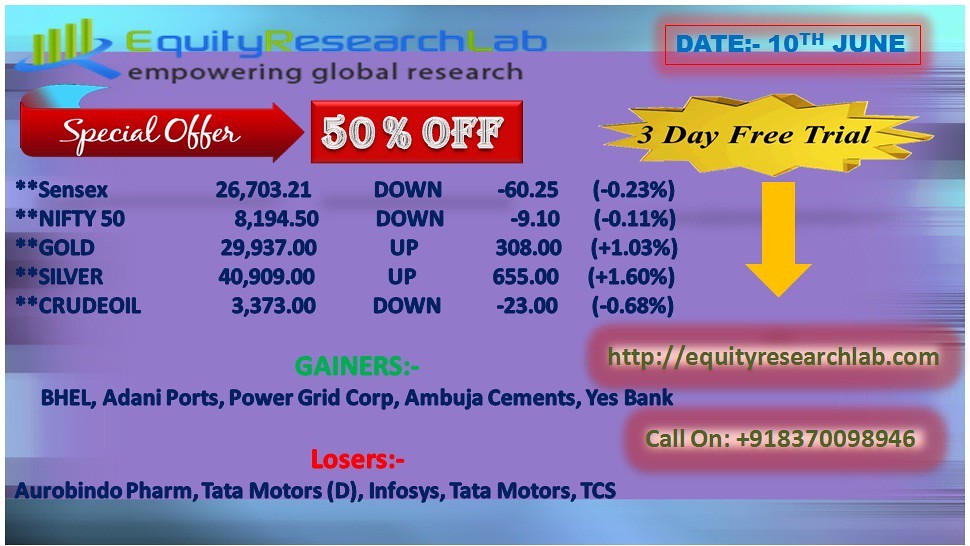The image is a detailed advertisement for a stock trading or suggestion service called Equity Research Lab, set against a predominantly purple background with lighter blue accents at the top and bottom. In the top left corner, the text "Equity Research Lab" is prominently displayed, followed by the tagline "Empowering Global Research." The top right corner indicates the date, "10th June," and highlights a "Special Offer: 50% Off." Below this, there's information about market indices and commodities, including "Sensex: 26,703.21, down -60.25 (-0.23%)," and "Nifty 50: 8,194.50, down -9.10 (-0.11%)."

Further details list the performance of various commodities: "Gold: 29,937, up +308 (+1.3%)," "Silver: 309, up +655 (+1.60%)," and "Crude Oil: 3,373, down -23 (-0.68%)." A table labeled "Gainers" in green includes stocks like "BHEL, Adani Ports, Power Grid Corp, Ambuja Cements, Yes Bank," while a "Losers" section notes "Aurobindo Pharma, Tata Motors D, Infosys, Tata Motors, TCS." 

On the right side, the advertisement mentions a "3-Day Free Trial" and provides an email address, phone number, and the company's website: "http://equityresearchlab.com" with the phone number "1-183-700-98946."